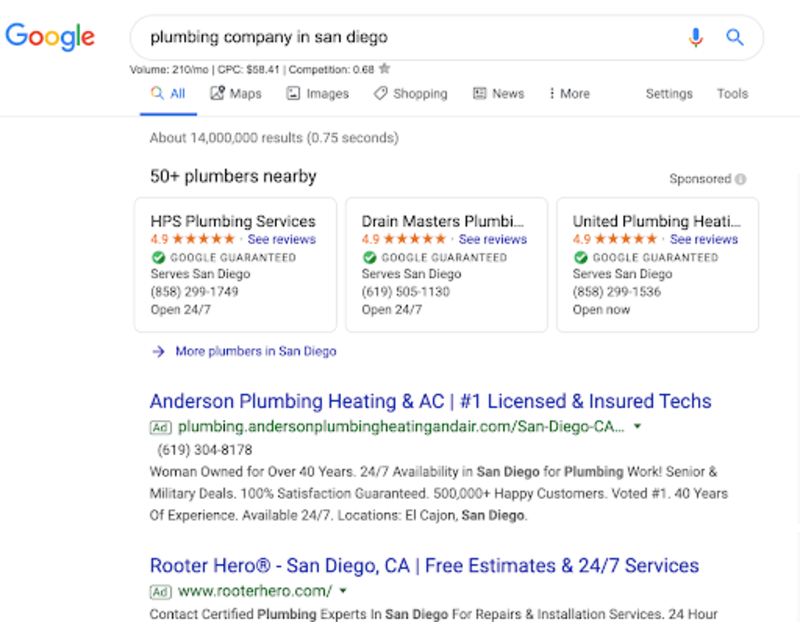This image depicts a screenshot of a Google search for "plumbing company in San Diego." In the upper left corner, the Google logo is displayed prominently in its iconic rainbow colors. Below the logo is the search bar containing the search query "plumbing company in San Diego." The user has clicked on the "All" tab, which is highlighted in blue with an underlined magnifying glass icon. 

The search results indicate that there are "50+ plumbers nearby." Below this heading, three prominent boxes showcase different plumbing companies. From left to right, they are: "HPS Plumbing Services," "Drain Masters Plumbing," and "United Plumbing and Heating." 

Further down, the image displays sponsored advertisements. The first ad is for "Anderson Plumbing, Heating and AC," which is identified as being licensed, insured, and highly rated (#1). The green "Ad" label is visible next to the URL "andersonplumbingheatingair.com" for San Diego, CA. The second advertisement is for "Rooter Hero," which offers free estimates and 24/7 services. This ad also features a green "Ad" label and a box surrounding it, with the URL "www.rooterhero.com" highlighted in blue.

Additional search results continue below these advertisements, marking the end of the visible portion of the screenshot.